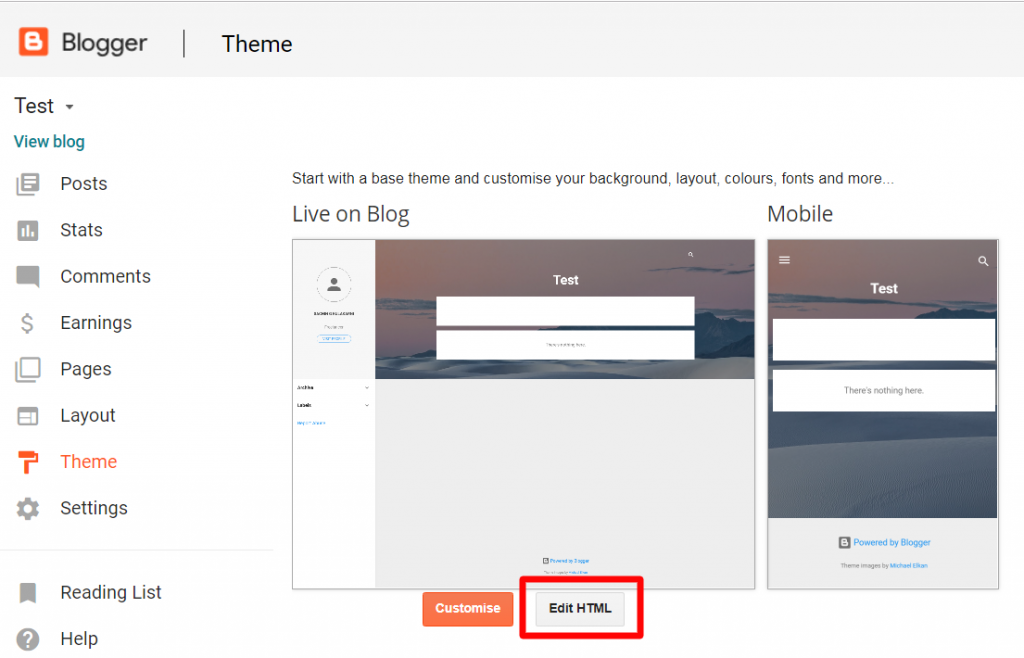The image is a screenshot from a Blogger website, where the user is in the process of selecting and customizing a theme for their blog. At the top of the page is a gray navigation bar that reads "Theme" prominently. There is a dropdown menu next to the word "Test," which is also labeled "View Blog" and colored blue. Below the navigation bar, there is a series of tabs labeled: "Post," "Stats," "Comments," "Earnings," "Pages," "Layout," "Theme" (highlighted in orange), and "Settings," with all tabs except "Theme" being in black text.

On the right side of the screen, there is a section titled "Start with a base theme and customize your background, layout, colors, fonts, and more." It also mentions that changes will be shown live on the blog. Below this section, there are two buttons: an orange "Customize" button and a gray "Edit HTML" button, with "Edit HTML" encased in a red outline. Additionally, the screen includes a preview of the blog’s mobile version, labeled "Test" at the top and "Powered by Blogger" with "Themes, images by Michael" at the bottom in blue text.

The website layout appears basic with site navigation elements displayed, featuring a placeholder for a photograph and spaces designated for writing content. The overall design of the page underscores a user-friendly interface for personalizing the blog's appearance.